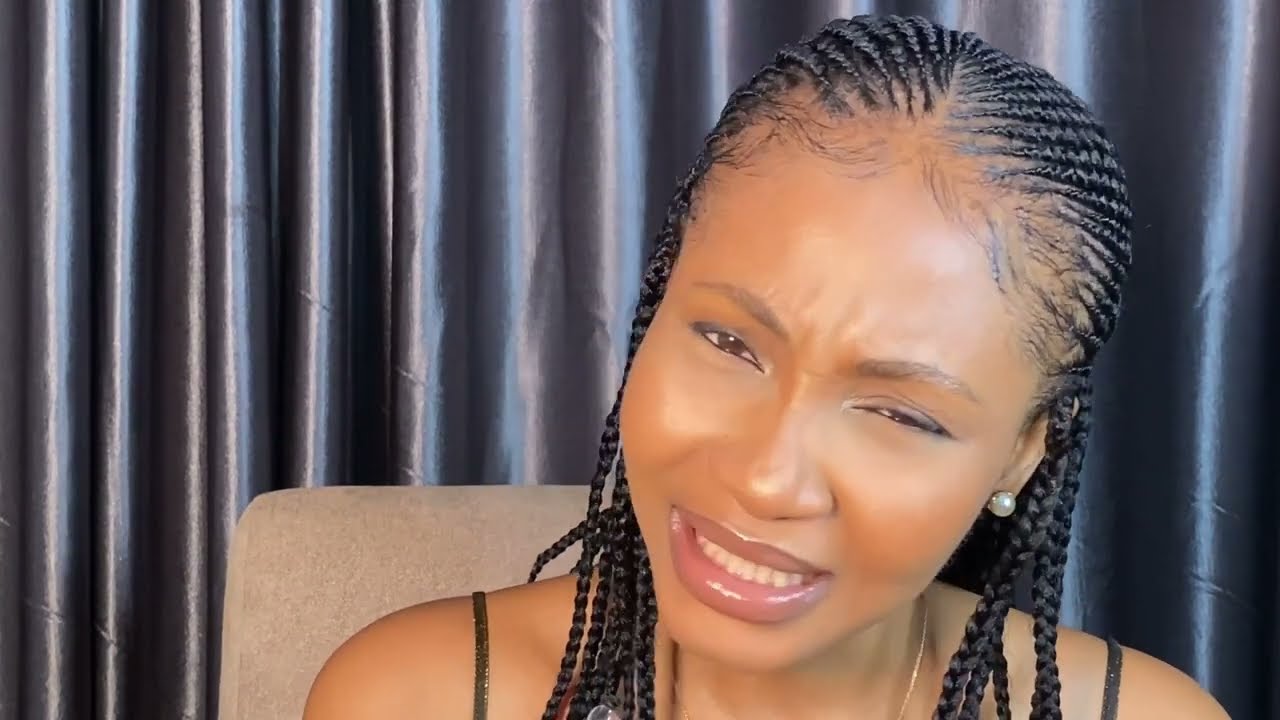This color photograph captures a young black woman from the shoulders up, positioned slightly to the left. She tilts her head to the right, her eyes squinting, and her mouth open as if speaking, revealing her teeth. Her neatly braided, black hair cascades around her bare shoulders, adorned with the thin black straps of a tank top. A single pearl earring dangles from her left ear. She occupies a beige chair, partially visible over her left shoulder, set against a pleated silvery-gray curtain that shimmers in the background. The lighting emphasizes her forehead, adding intensity to her appearance. Her glossy lips, combined with the various hues in the image—including shades of brown, pink, white, deep navy, and dark purple—suggest she might be engaged in an online video chat, possibly from a home setting like a bedroom, living room, or home office.